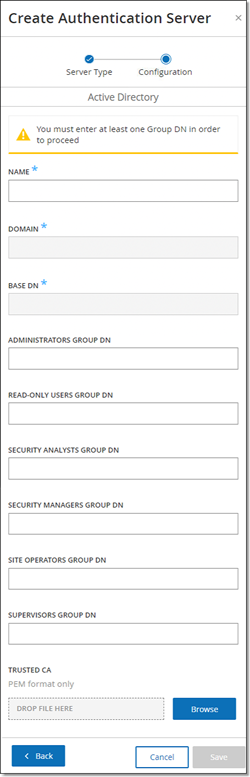Screenshot depicting a mobile application interface for creating an authentication server. The interface is displayed in a narrow window with a white background enclosed by a dark gray or black border. 

At the top of the window, in bold black text, is the title "Create Authentication Server". To the right, a light gray 'X' allows users to close the window. A gray horizontal line separates the header from the main content.

Below the line, a progress indicator features a blue dot with a white check mark on the left, labeled “Server Type,” connected to another blue dot with a darker blue center on the right, labeled “Configuration,” by a horizontal gray line.

Following another gray line, the text “Active Directory” is displayed in light gray large lettering, under which another gray line appears. Below this, a lightly outlined gray box contains a yellow strip at the bottom and a yellow triangle with a white exclamation mark on the left, signaling a warning: "You must enter at least one group DN in order to proceed".

The form below the warning contains text boxes with the following labels, all marked with black text and a blue star indicating required fields:
- Name
- Domain (not filled in)
- Base DN (not filled in)
- Administrator’s Group DN (not filled in)
- Read-Only Users Group DN (not filled in)
- Security Analysis Group DN (not filled in)
- Security Managers Group DN (not filled in)
- Site Operations Group DN (not filled in)
- Supervisors Group DN (not filled in)
- Trusted CA (with light gray text indicating “PEM format only”)

A gray search bar beneath these fields contains the text “Drop file here” and a blue "Browse" button in white text to its right. At the bottom left of the window, a blue button with white text reads “Back”, next to a outlined blue button with blue text on a white background that says “Cancel”. On the far right, a gray button with white text reads “Proceed".